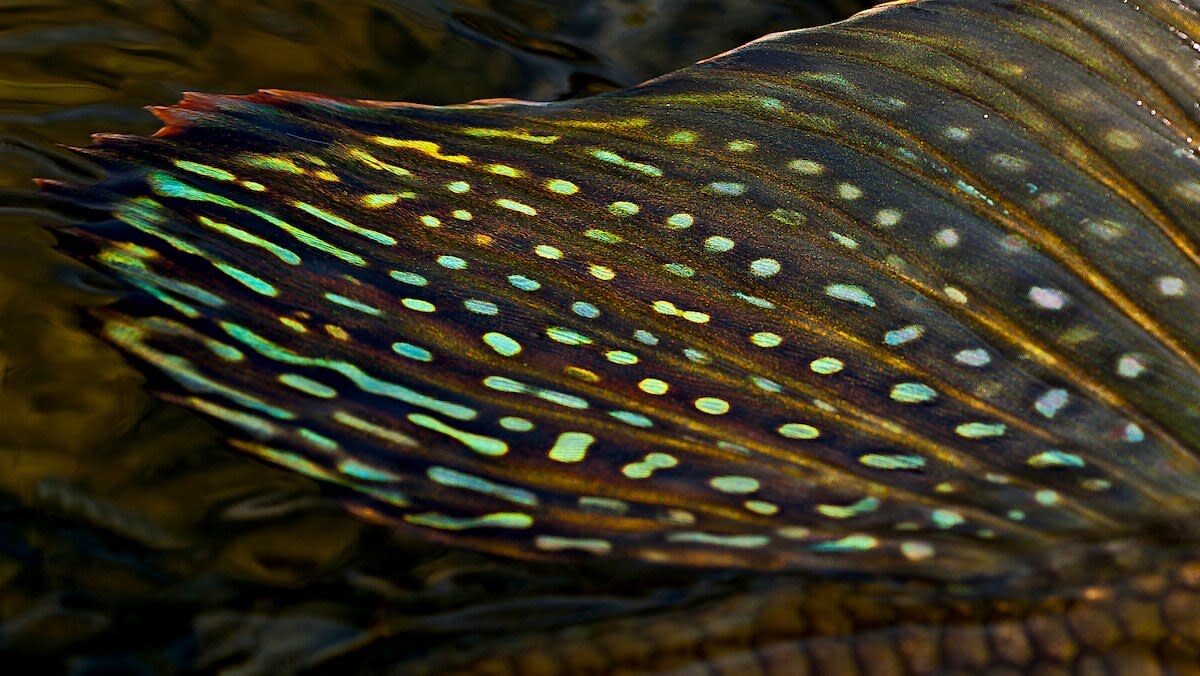The image depicts a close-up of a butterfly wing, characterized by intricate and vibrant details. The wing is adorned with yellow, green, and blue dotted patterns, interspersed with red tips at the far end, suggesting these features contribute to the overall complexity and beauty of the wing. The background of the photograph is dark, which makes the bright, intricate design stand out more strikingly. Along the bottom section of the wing, there appear to be scaly, yellowish-brown segments, resembling the segmented patterns found in butterfly wings, particularly reminiscent of a monarch butterfly, albeit with a different color palette. The wing itself has a heart-shaped appearance, with brown edges transitioning into the center from left to right, adding to its unique structure. The combination of these elements creates a vivid and detailed portrayal of the wing's natural patterns and textures.